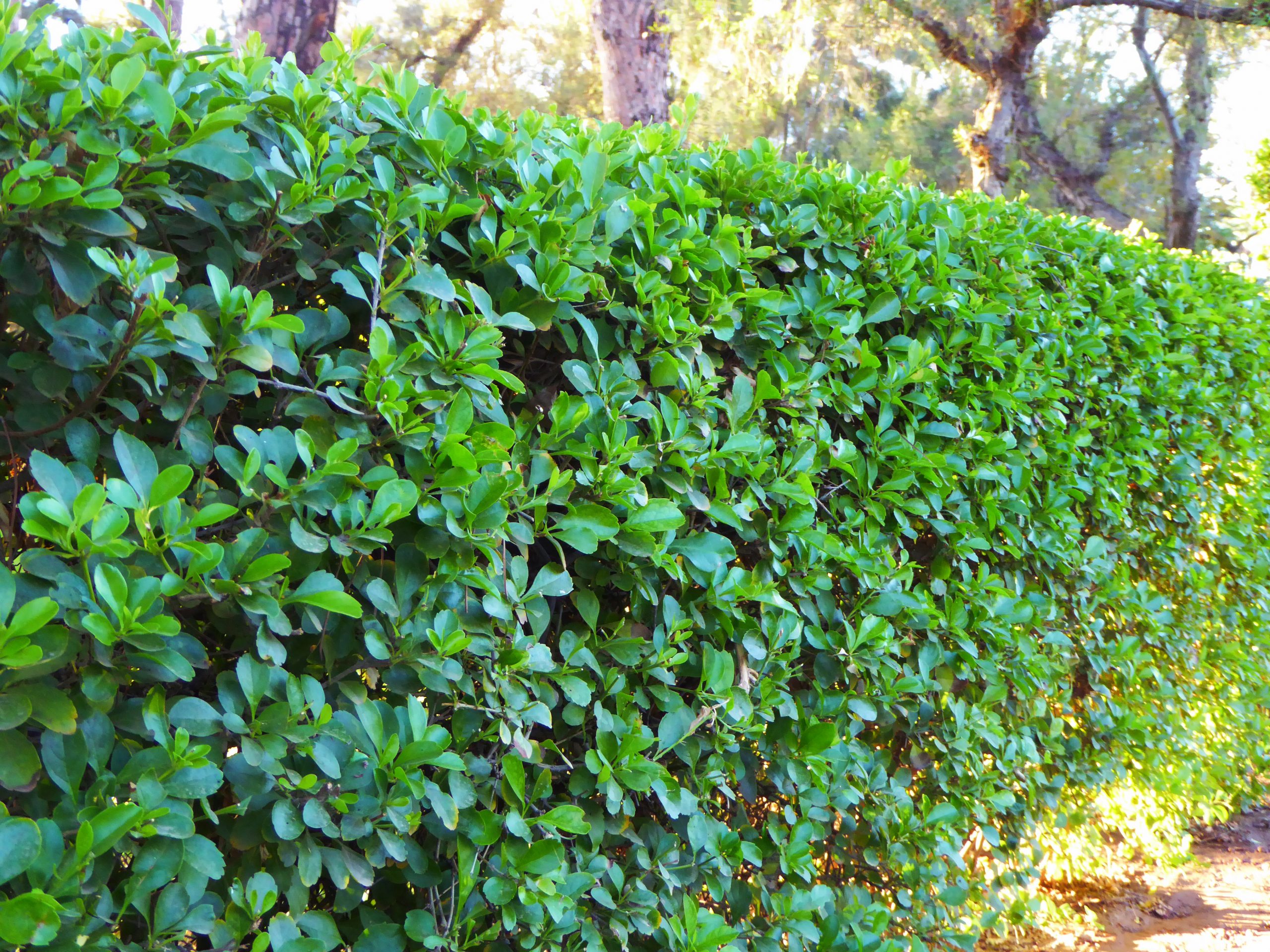The photograph is an up-close, vibrant capture of a neatly manicured green hedge, revealing a uniform layer of small, round leaves. The hedge runs across the entire length of the image, making it difficult to determine where it begins or ends. Towards the bottom right corner, a patch of dusty ground with some yellowish leaves is visible, illuminated by the sunlight breaking through the foliage. Above the hedge, the background features larger trees and their upper trunks, slightly out of focus, with sunlight filtering through the branches. Hints of the sky, appearing almost white, are visible amidst the trees, suggesting a bright, sunny day.